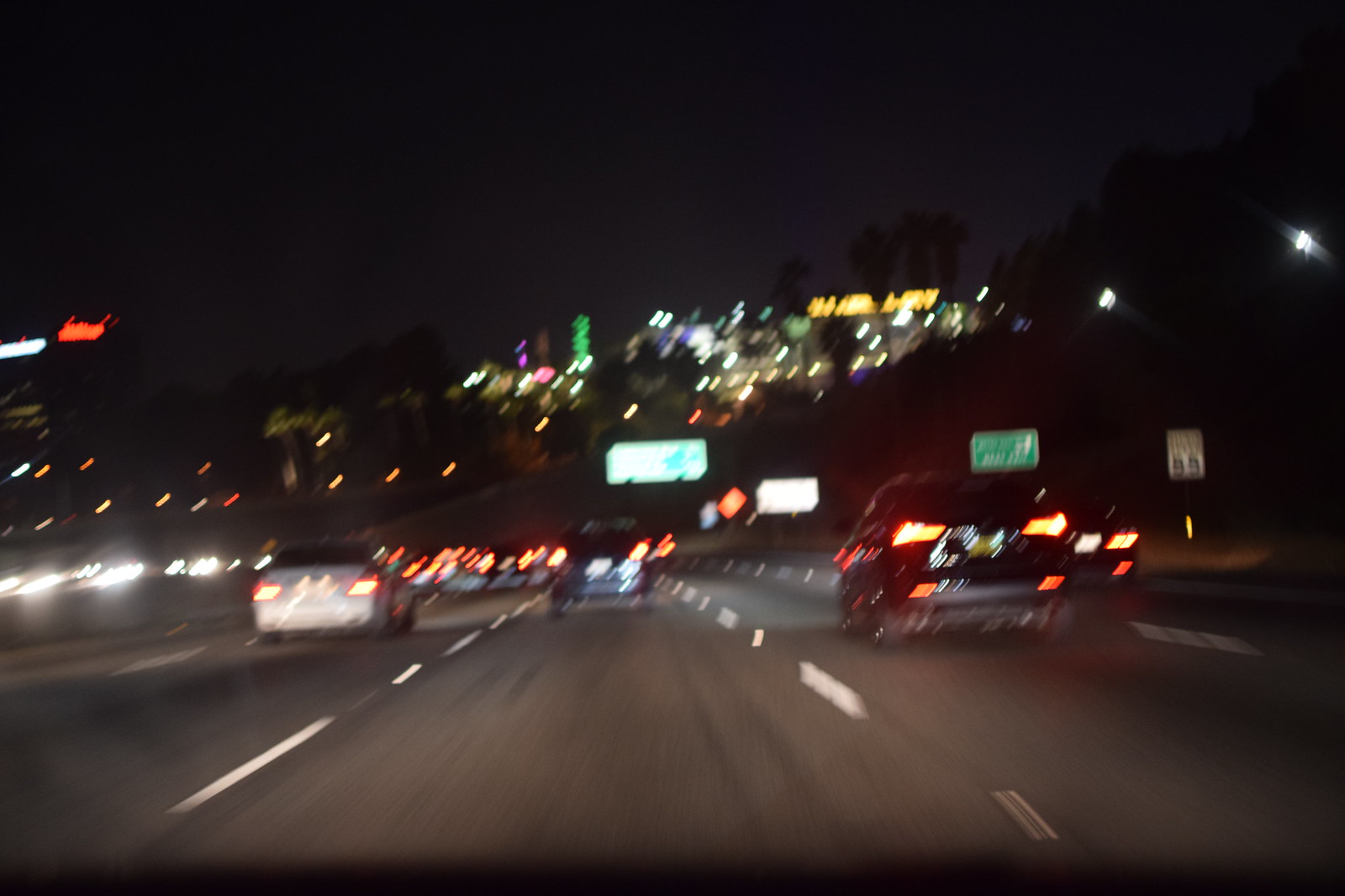The image shows a nighttime view captured from inside a moving vehicle on a large freeway, taken through the windshield. The freeway comprises at least five lanes of northbound traffic, with numerous cars visible ahead, their taillights forming a blurred trail due to the vehicle's motion. On the opposite side of the freeway, headlights from southbound traffic shine brightly. Up ahead, there is a cluster of colorful lights—greens, purples, yellows, and whites—suggesting proximity to a city. Street signs are visible in the distance, with one indicating a speed limit of 55 miles per hour. The overall scene is bathed in the ambient glow of urban illumination, accentuated by the blurriness that emphasizes the sense of motion.